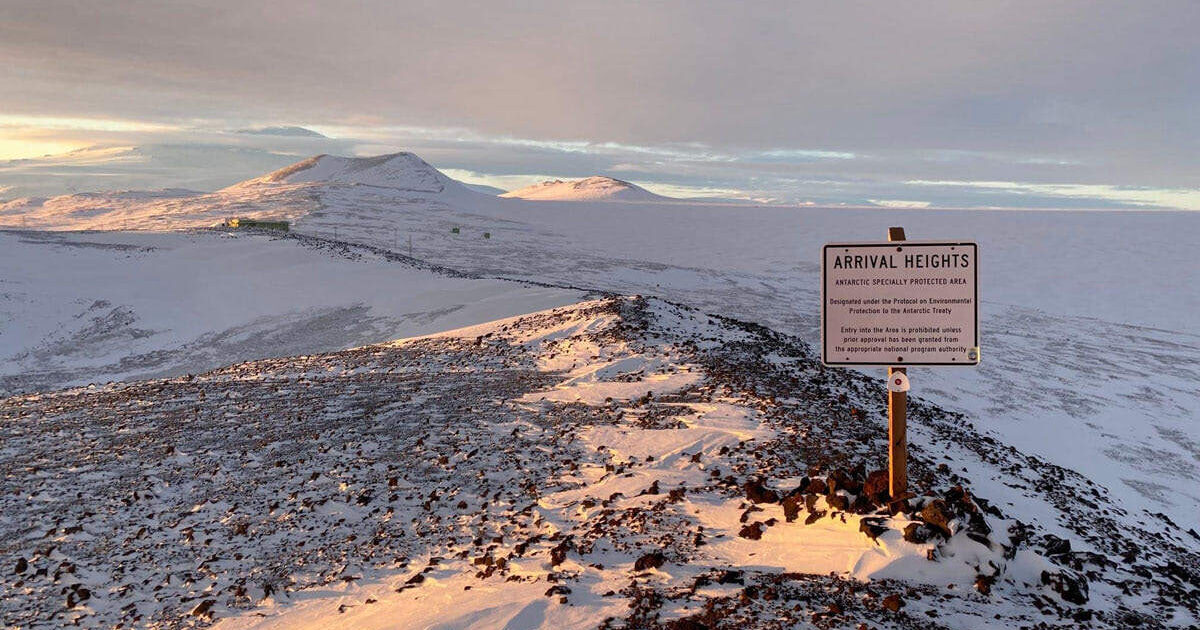This is a detailed landscape photograph capturing the stark beauty of a snowy mountain peak in a sideways orientation. Dominating the foreground is a white sign with black lettering fixed on a wooden post, declaring: "Arrival Heights, Antarctic Specially Protected Area," followed by several unreadable lines. The area appears desolate and uninhabited, with scattered rocks protruding through the snow. The background unfolds into a vast and expansive mountain range, with three distinct peaks visible in the distance. There’s a hint of a small unidentified structure further back, adding to the photograph's sense of isolation. The sky above is heavily blanketed with clouds, evoking a cold, blue, and almost melancholic atmosphere, as if foretelling an imminent snowfall. The entire composition exudes a tranquil, yet forbidding, allure.